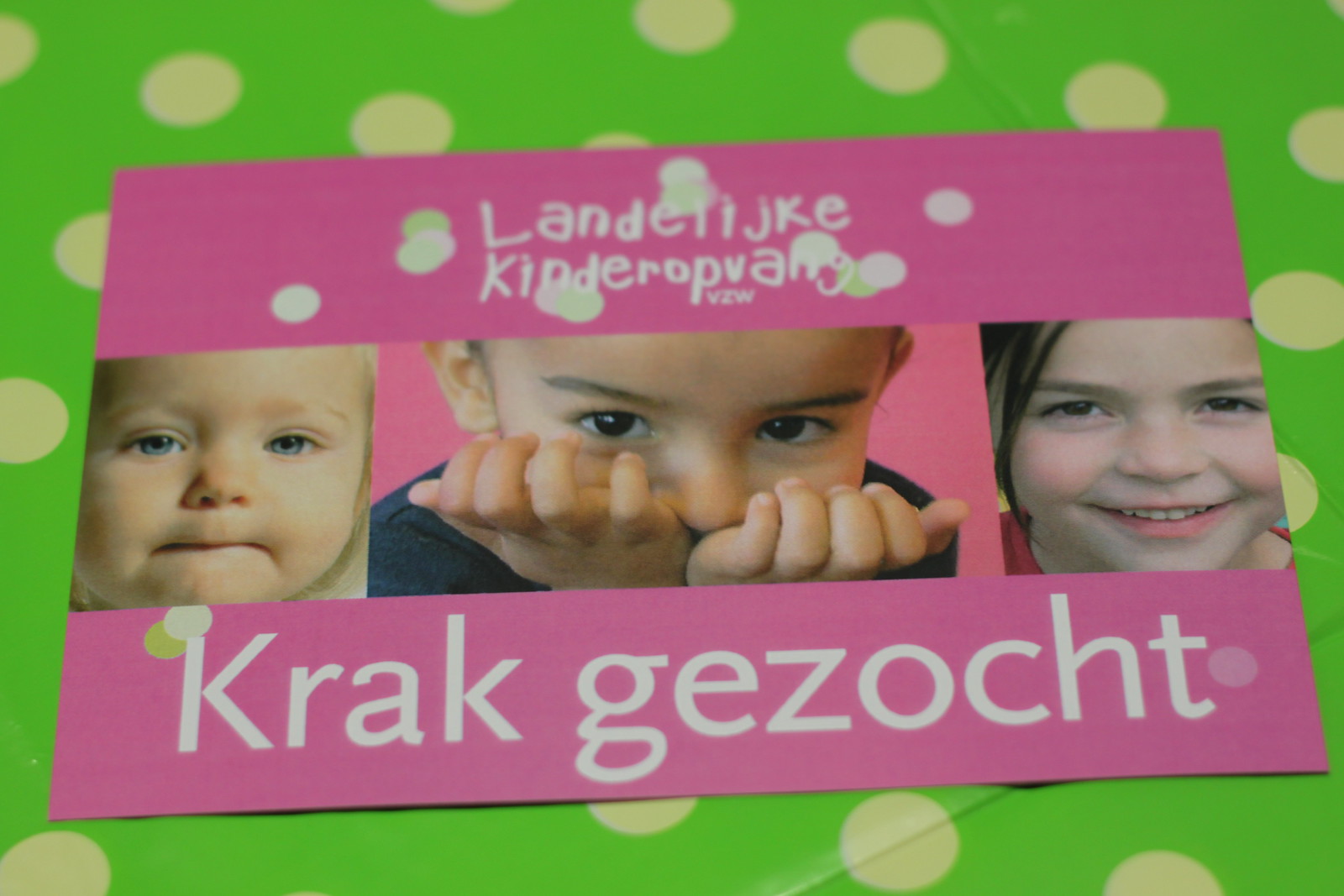The image depicts a postcard-style advertisement with a detailed and colorful design. The background consists of green with yellowish polka dots. The postcard itself is pink and features three images of children positioned side by side in the center. The child in the middle is a blonde girl with blue eyes and a pursed mouth, while the boy on the left has dark brown eyes and covers his mouth with his hands, and the girl on the right has brown hair, brown eyes, and is smiling at the camera. The postcard also has polka dots in purple, green, and yellow on its pink background. The text on the card is in a foreign language, possibly saying "Lend-A-Leek Kinderop," with the top text in a playful, loopy font and the bottom text in a straight font. The entire setup suggests it is an advertisement for a kindergarten or a children's program, based on the visual elements and context provided. The image is laid on a possibly flat surface such as a table or cloth.